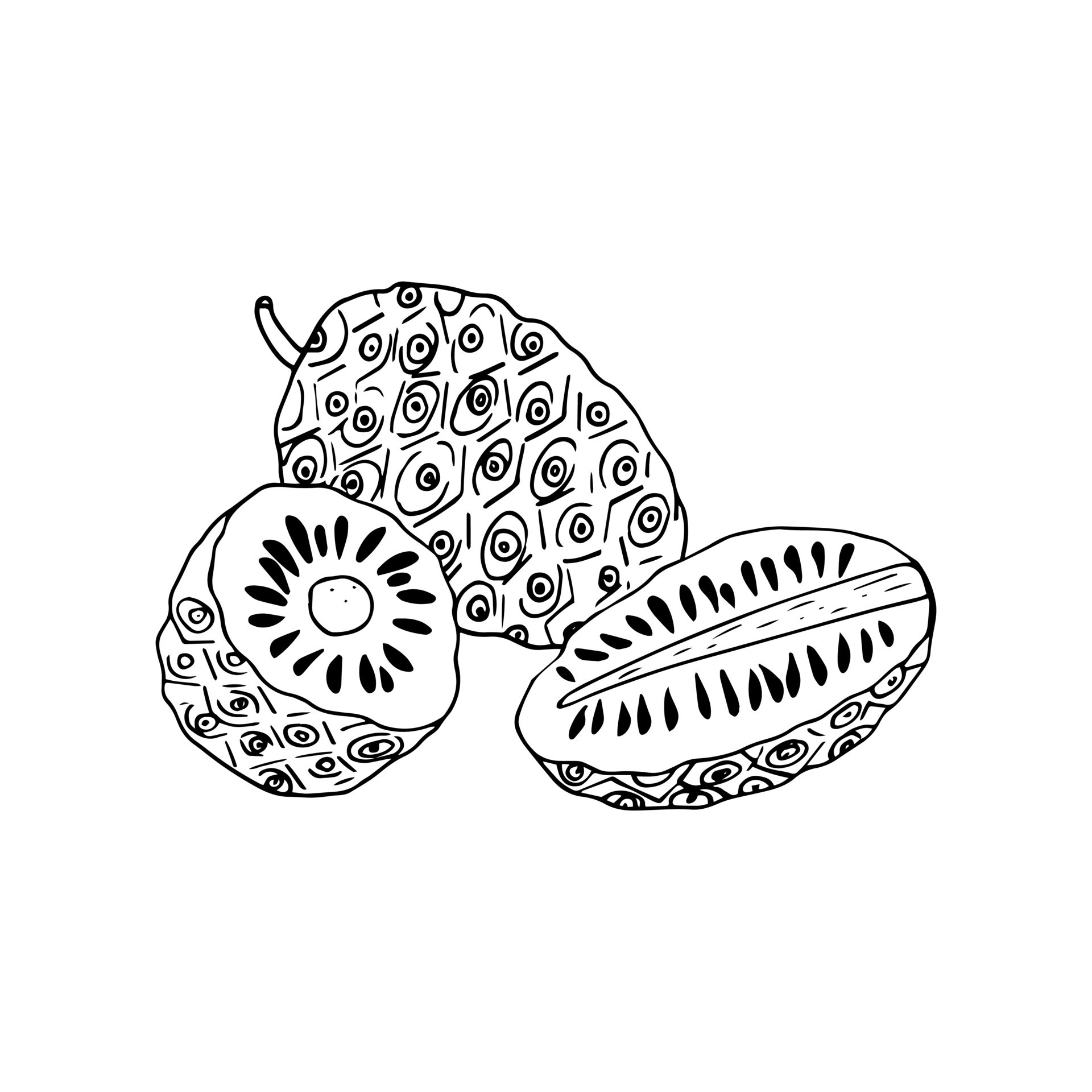This black-and-white, pen-and-ink drawing features three detailed, stylized depictions of a fruit. In the background, the whole fruit is drawn with a stem on its upper left side, showcasing an oval shape with intricate, textural details consisting of circles, ovals, and straight lines. In the foreground, the fruit is artistically presented in two different sections: one cut lengthwise, and the other in a cross-sectional, circular shape. Both cuts reveal the fruit's interior features, including a central pit surrounded by numerous small, round seed-like objects. The intricate design and textured techniques provide a unique, art-based interpretation of this unidentified fruit.